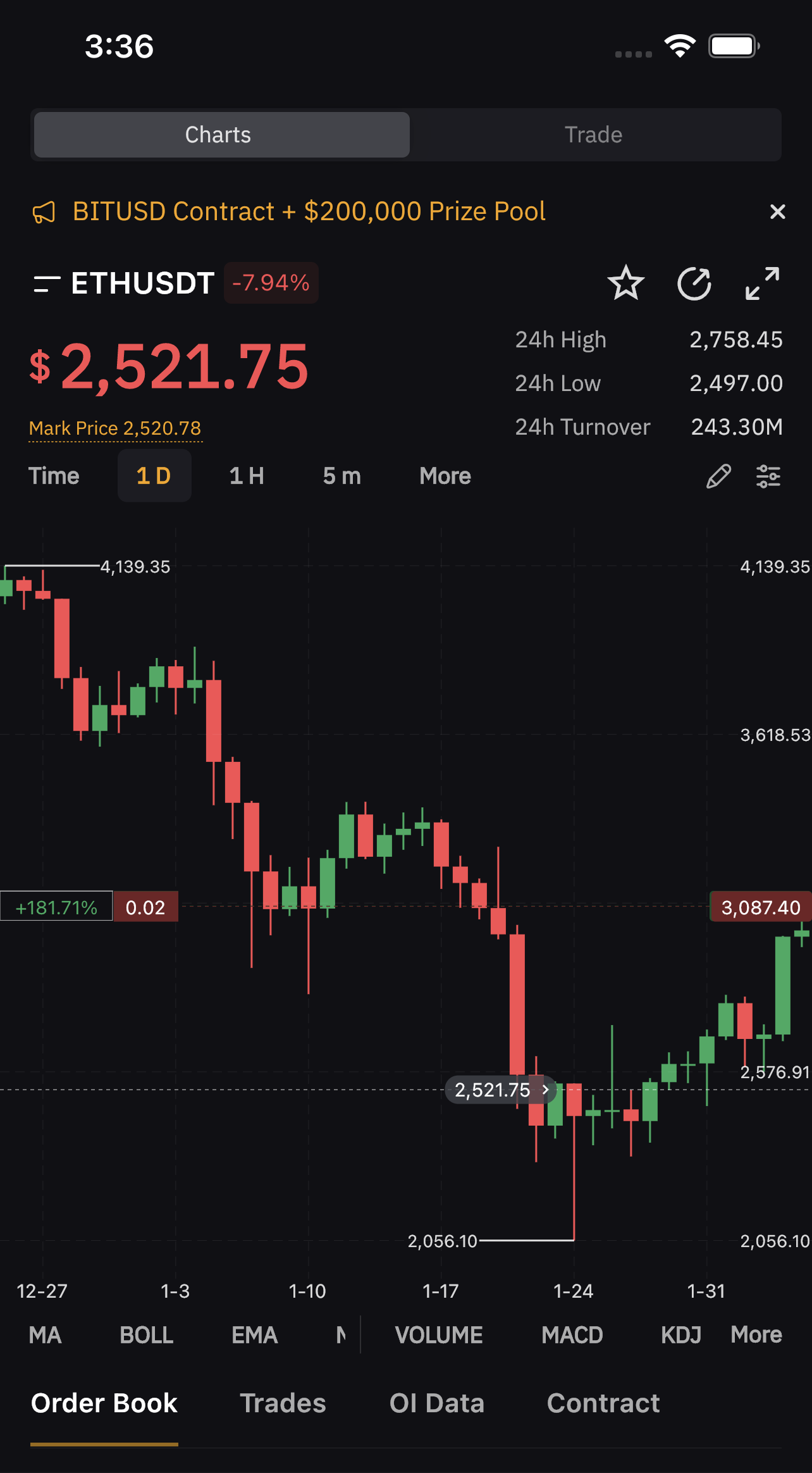A detailed screenshot of a cryptocurrency tracker application displays a wealth of information on a black background with white text. 

In the upper left-hand corner, the time is displayed as 3:36. Opposite, in the upper right-hand corner, icons indicate a full Wi-Fi signal and a fully charged battery. Directly below these indicators are two tabs: "Charts" and "Trade," with "Charts" highlighted.

Central to the screen, a banner reads "BITUSD contract + $200,000 prize pool." Immediately following, the text "ETHUSDT" is displayed in white, with a negative value of -$7.94 in red text below it. Dominating the center of the screenshot, a large red figure, $2,521.75, indicates the current value or a significant metric for ETHUSDT.

Beneath this, a bar chart with black and green lines visually represents market data over a specified time period. The chart is annotated with white labels for various statistical indicators, such as MA (Moving Averages), BOL (Bollinger Bands), MA Volume, KDT, among others, providing detailed financial insights.

Further down, options are available for viewing open book trades, OI (Open Interest) data, and contract details, offering a comprehensive overview for the user. The entire interface maintains a professional aesthetic with its black background and high-contrast text, ensuring clarity and a focus on critical financial information.